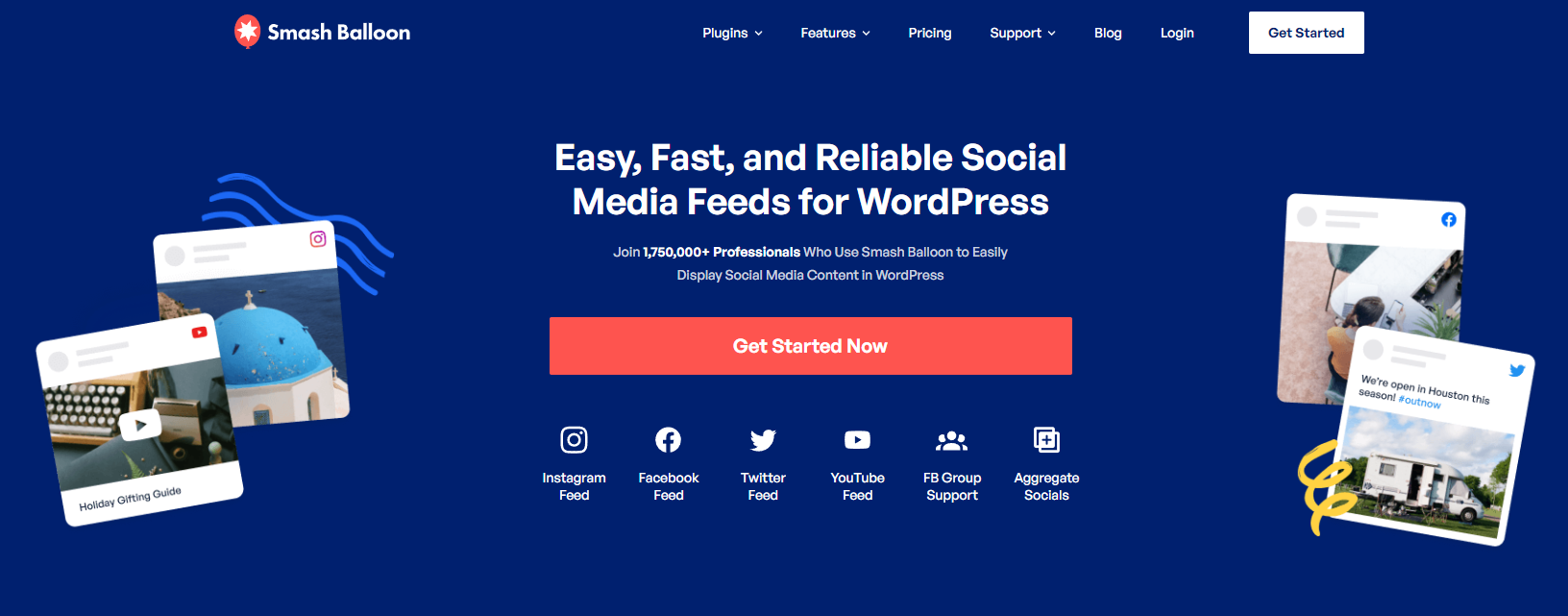This is a detailed caption for the image described:

---

This is a webpage from Smash Balloon featuring a prominently dark blue background. At the top of the page, there is a navigation bar with tabs labeled "Plugins," "Features," and other options including "Support," "Login," and "Get Started." The "Get Started" button is distinctively set in a white box with blue lettering.

To the left side of the page, there is an embedded video showing real-life photography. Above the video, there's an orange circle with a white interior resembling a floral design.

In the main content area, centered text declares, "Easy, Fast, and Reliable Social Media Feeds for WordPress" in white font. Below this headline, smaller print provides additional details. Directly beneath, another "Get Started" button is positioned, flanked by icons representing Instagram, Facebook, Twitter, and YouTube.

Just below, there is mention of a Facebook support group, and another section characterized by icons of two boxes joined by a plus sign, although the text here is not completely legible.

To the right side of the screen, the page displays two additional images. One depicts a camper, and the other shows a person working at a lengthy desk. Both add to the visual narrative of the webpage.

---